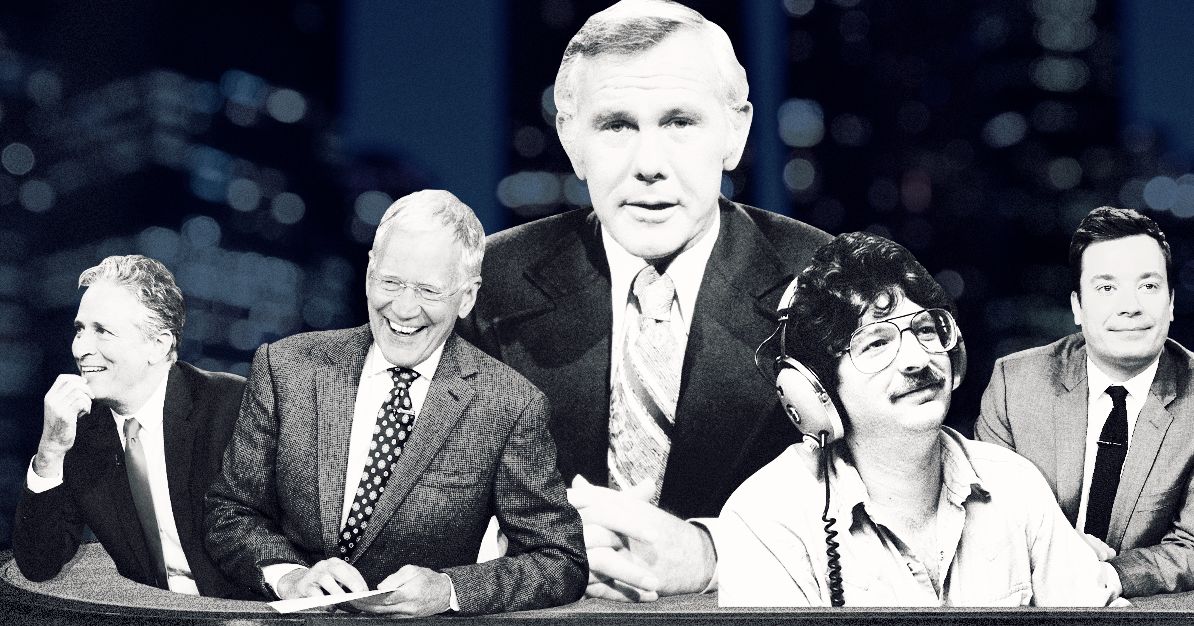The image is a meticulously photoshopped black-and-white composite featuring five prominent late-night talk show hosts against a blurred skyline of skyscrapers. Dominating the center is the iconic Johnny Carson, seamlessly presented in a sharp, stoic pose with his hands folded, embodying the essence of his 'Tonight Show' persona. To his right are smaller images of David Letterman, holding a paper and laughing, and Jon Stewart, both exuding their signature charisma. On Johnny's far left is Jimmy Fallon, recognizable in a dark tie and suit, subtly maintaining his comedic poise. In the foreground, on Johnny's lower left, sits an unidentified man wearing large, vintage over-the-ear headphones and big-rimmed glasses, possibly from the seventies or eighties, with thick, black curly hair and a voluminous shirt. The detailed arrangement and varying expressions emphasize the disparate eras and styles, underscoring the surreal nature of this digitally created assembly.